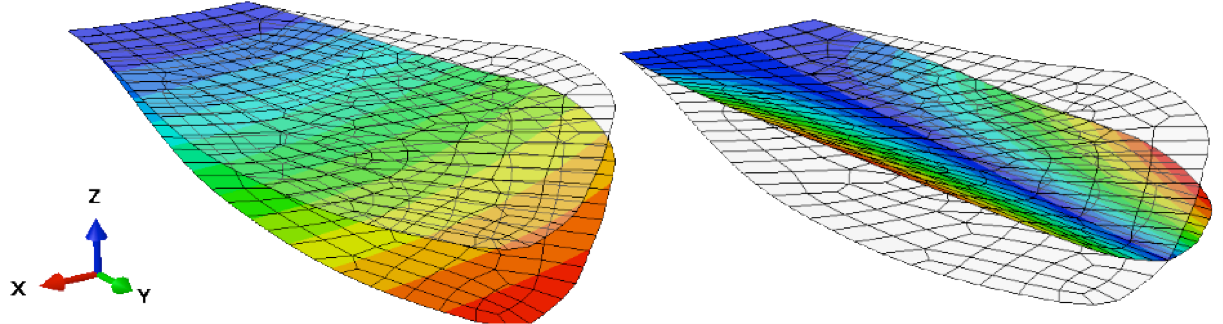The image features a white background with two distinct three-dimensional topographical maps or graphs. These maps are adorned with a spectrum of colors including blue, teal, green, yellow, orange, red, and purple, forming distinct stripes and patterns. Each map is overlaid with a grid of rectangles, creating a mesh-like appearance. 

To the left of the maps is a legend that includes three arrows labeled with letters indicating directions: a blue arrow pointing upwards labeled "Z," a red arrow pointing to the bottom left labeled "X," and a green arrow pointing to the bottom right labeled "Y." One of the maps prominently features more white areas beyond the rainbow colors. The intricate detailing and spectrum of colors suggest these are digital 3D surface representations, showcasing different angles or data types.